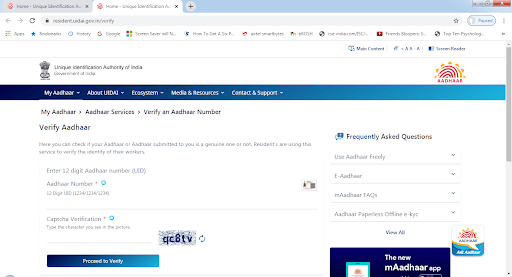This image displays a webpage from the Unique Identification Authority of India (UIDAI) with two browser tabs open. 

At the top right corner, there is an icon resembling a sun, accompanied by the text "Adhemar." To its left, the title "Unique Identification Authority of India" is prominently displayed. Below the title, a blue navigation bar contains various links including "My Adhemar," "About Us," "Ecosystem," "Media Resources," and "Contact and Support."

Further down, the page is structured as follows: 
- A header labeled "My Adhemar" leading into options like "Aadhaar," "Aadhaar Services," and "Verify an Aadhaar Number."
- The section "Verify Aadhaar" contains instructions and a text box labeled "Enter 12-Digit Aadhaar Number" for users to input their Aadhaar number.
- Adjacent to this field is a "Captcha Verification" section with an alphanumeric Captcha box that needs to be completed.
- A blue "Proceed to Verify" button is available for users to click once they have filled in the necessary details.

On the right side of the page, there is a "Frequently Asked Questions" section with subsections such as "Use Aadhaar Freely" and other fields that are hard to decipher. Additionally, a prominent blue box advertises "The New M Aadhaar App," encouraging users to explore this feature.

The overall layout is detailed and focuses on facilitating the verification of Aadhaar numbers while providing easy access to additional resources and support.